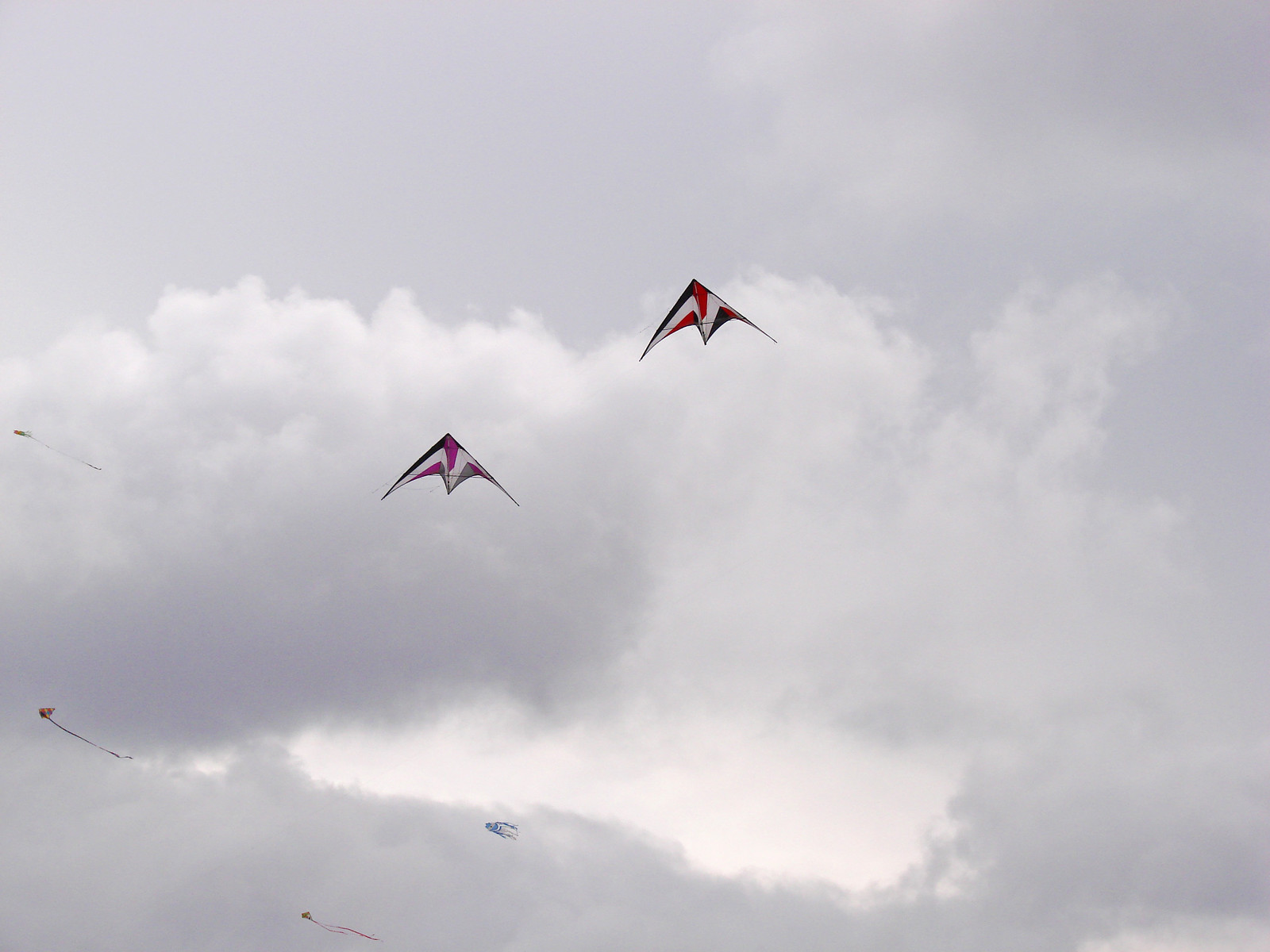In this photograph of an overcast sky filled with puffy gray and white clouds, we see six kites soaring high. The image is captured from below, facing upwards toward the cloudy sky. Two prominent kites, triangular with arched curves resembling an 'M' or bat-like shape similar to a Batman icon, stand out. These kites display a geometric design in shades of pink, white, black, red, and blue. The red appears at the top, followed by white, with blue edging at the bottom. One of these kites, slightly lower and to the left, is paired with another higher up to the right. Smaller kites populate the background, including one distinct kite shaped and styled like a blue and white fish. The scene is bright, despite the overcast, and the smaller kites' details become faint due to their distance.